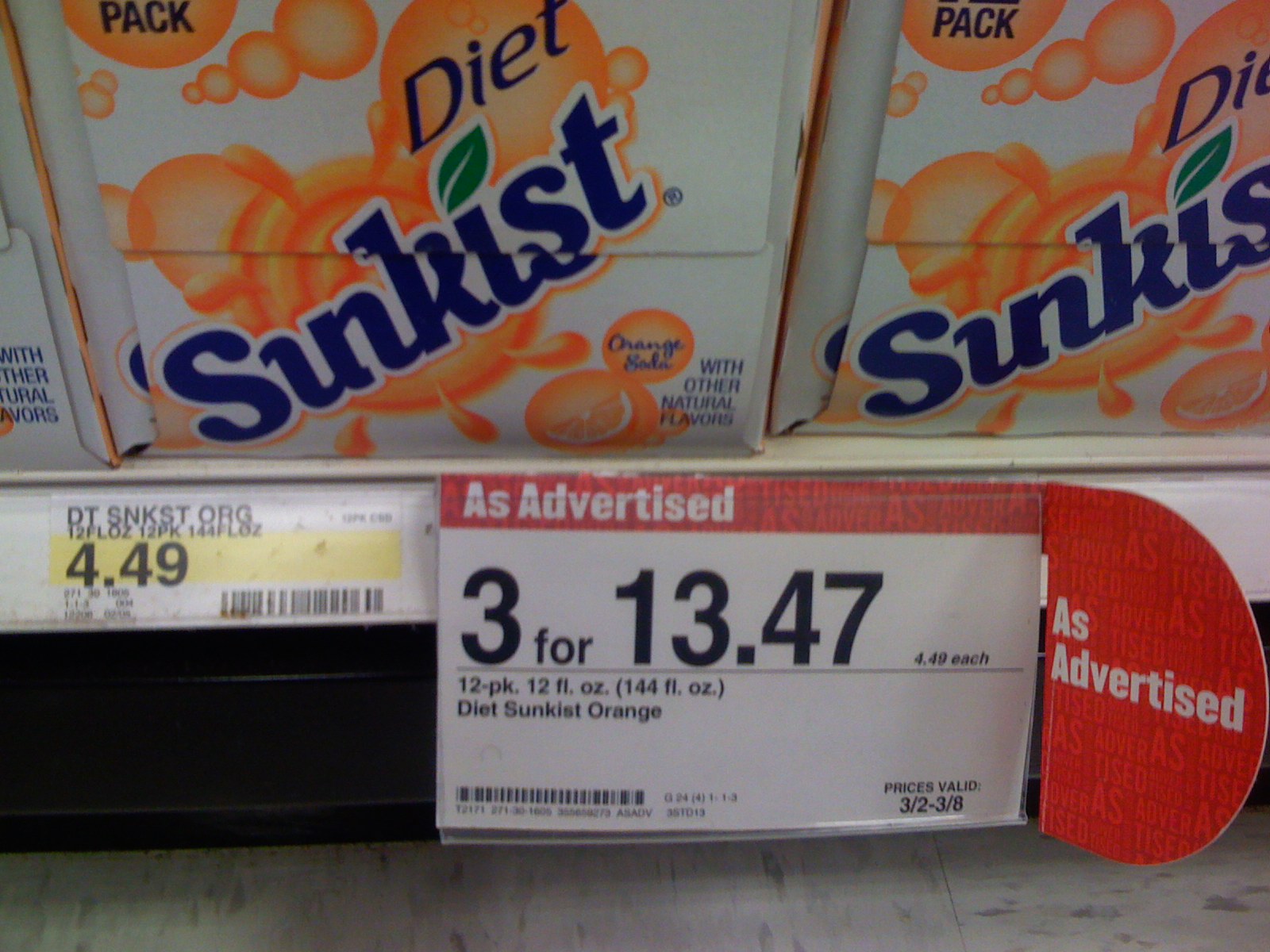In this photograph, taken inside a Target store, the viewer is looking down at the bottom shelf in the soda aisle. Prominently displayed are 12-pack cases of Diet Sunkist Orange soda, each containing twelve 12-fluid-ounce cans, totalling 144 fluid ounces per pack. The price tag visible on the shelf indicates each 12-pack is priced at $4.49. Additionally, there is a promotional sign above the cases that reads "As Advertised: 3 for $13.47," suggesting a bulk deal valid from March 2nd to March 8th. The image details the precise arrangement and pricing of the product within a typical store setting.